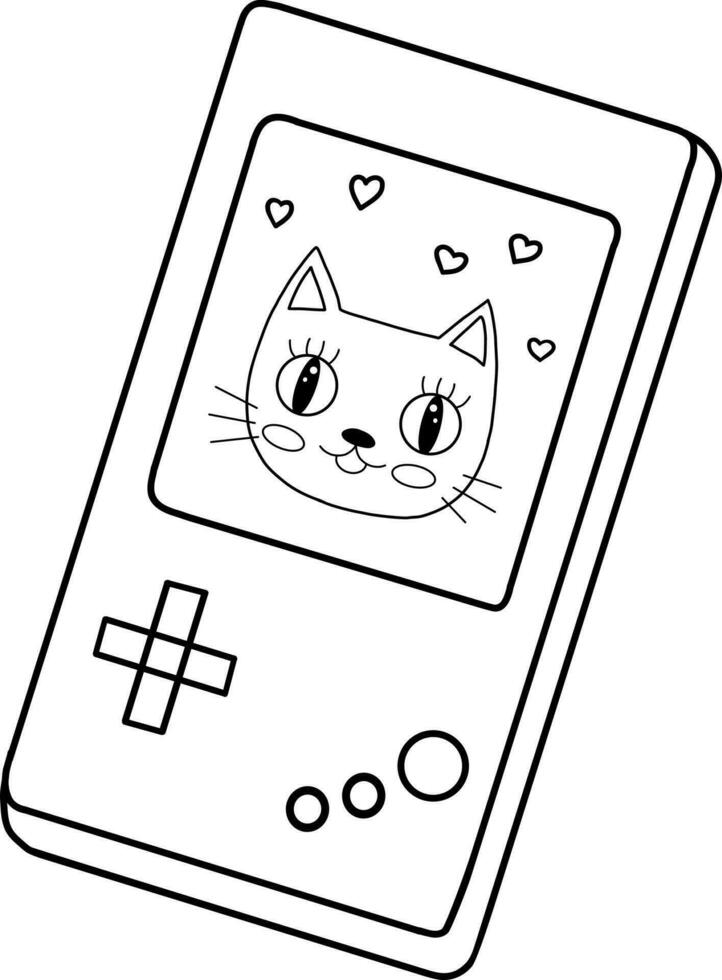A simple, black-and-white illustration of a retro Game Boy-like device, with a playful and child-friendly style reminiscent of a coloring book page. The device is a rectangular shape with rounded edges and a subtle 3D effect, set against a completely white background. The screen, also rectangular with rounded corners, features a cute cartoon cat face. This adorable cat has big eyes, a smiling face with its tongue playfully sticking out, and detailed features including whiskers, heart shapes floating around, and little ovals on its cheeks. Tiny triangles are drawn inside its ears, enhancing its endearing look. In the bottom left corner of the device, there is a cross-shaped arrangement composed of two intersecting rectangles and three small circular buttons, adding to the nostalgic design of the handheld device.